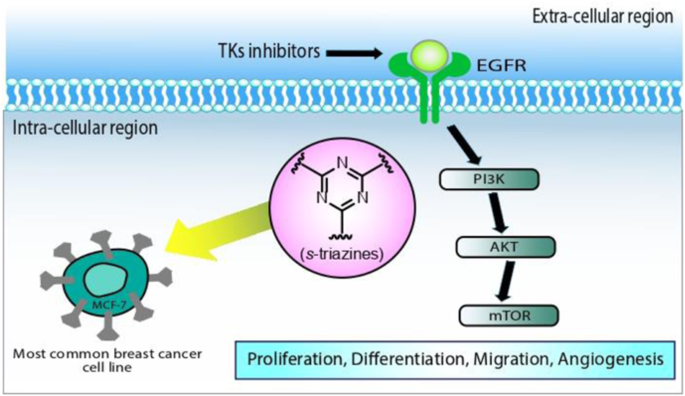This detailed infographic from a science book illustrates the signal transduction pathways associated with the most common breast cancer cell line, MCF-7. The image is divided into two main sections: the extracellular region, labeled at the top, and the intracellular region, labeled below a white, DNA-like double helix that spans the width of the chart.

In the extracellular region, "TKs inhibitors" is prominently displayed with a black arrow pointing to a green sphere held by two green, claw-like structures, labeled "EGFR." The EGFR complex penetrates the DNA-like boundary and continues into the intracellular region.

In the intracellular region, the MCF-7 cell is shown with a purplish-pink, diamond-shaped nucleus. The nucleus features a chemical diagram of a molecule identified as "S-triazines" in parentheses and depicted with three nitrogen rings. To the right, a series of black arrows point downward in a hierarchical manner, connecting boxes labeled "PI3K," "AKT," and "MTOR," representing a signal pathway. Below these, a light blue box lists the cellular processes affected by these pathways: "proliferation, differentiation, migration, and angiogenesis."

Additional details include labeled sections, a depiction of receptors on the MCF-7 cell, and various directional arrows indicating the flow of signals. This comprehensive illustration integrates cell biology with chemical annotations and molecular interactions relevant to breast cancer research.